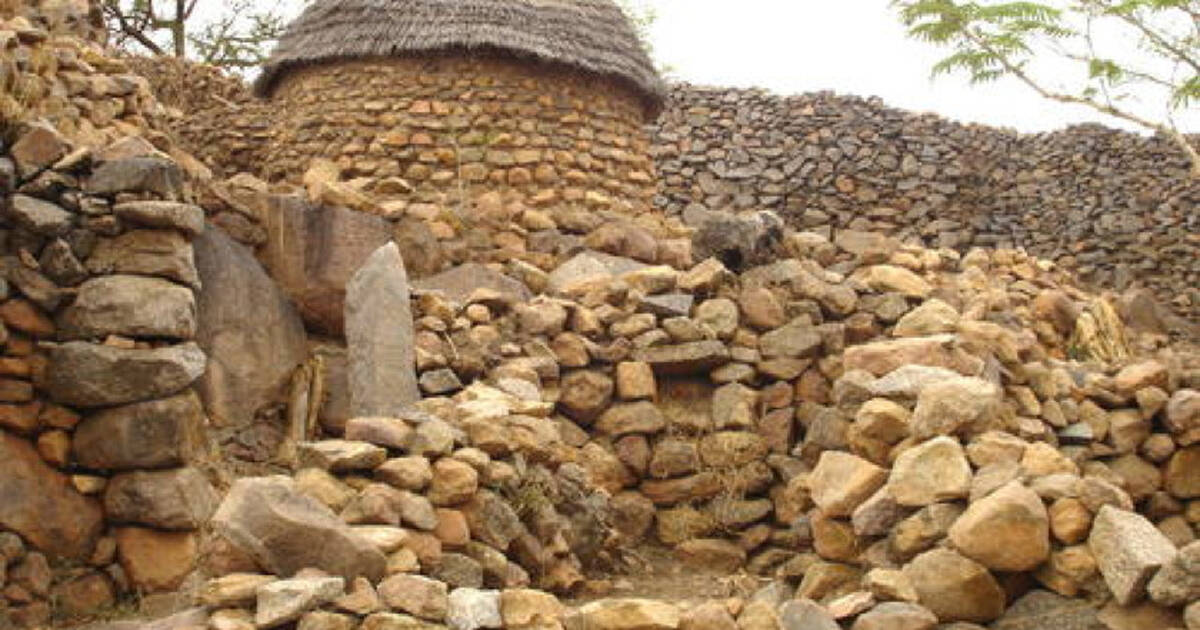The photograph captures the ruins of what appears to be an old, stone-built structure, possibly an African fort or hut. At the top of the image, a white sky serves as a backdrop, with tree branches sporadically piercing its expanse on both the right and left sides. Below this, a tan and gray stone wall stands out, its loosely stacked stones forming a rough, irregular surface. Dominating the center is a stone hut with a circular base and a thatched, straw roof, suggesting a traditional construction method. The midground features a more intact segment of the wall, showcasing larger boulders methodically incorporated amidst smaller stones. The foreground reveals a chaotic assemblage of tan and gray stones, some vertically stacked, larger on the left side compared to the right. These stones create a vague wall shape with a makeshift alcove-like structure. The stone walls appear to be built without mortar, with smaller stones wedged between larger ones for stability, hinting at an old, perhaps ancient, method of construction.